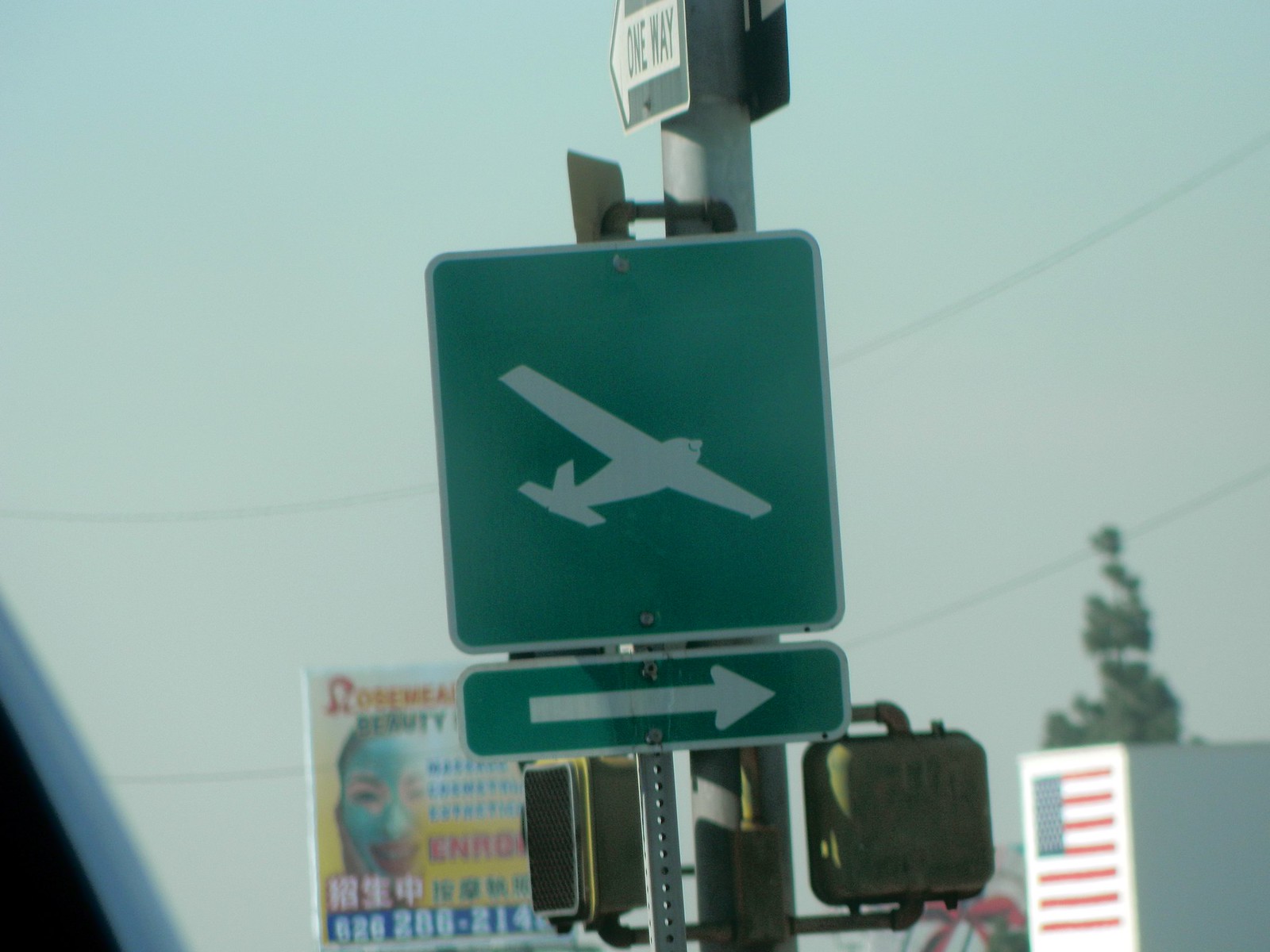This photograph, taken through a car window, captures a bustling street scene in Southern California, possibly Rosemead. Central to the image is a traffic pole adorned with multiple signs. At the forefront, there's a street sign featuring a white airplane icon, indicating the airport is to the right. Above it, a directional arrow reinforces the rightward direction. The pole also holds a one-way sign, along with electronic walk and don't walk signals. In the background, a large billboard prominently displays a woman's face wearing a mask, with text written in both English and Chinese, suggesting an advertisement for a spa. An American flag is visible on a nearby structure, adding a patriotic touch to the urban landscape.